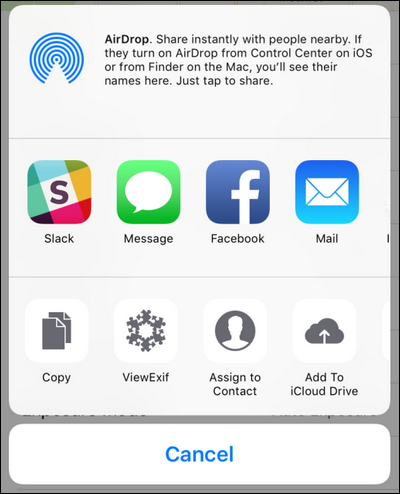An image is presented showing a user interface for sharing content across various platforms. The central text reads "AirDrop," accompanied by blue wing-like graphics around the corners. Beneath this heading, it instructs users to "Share instantly with people nearby. If they turn on AirDrop from Control Center on iOS or from Finder on the Mac, you'll see their names here. Just tap to share." The interface prominently displays the Slack app icon, distinguished by a blue "S" symbol. Several other icons are listed below, including various functionalities and applications:

- A green icon labeled "Speech" corresponding to the Messages app.
- The familiar Facebook icon, a blue square with a white "F."
- The Mail app, signified by a square icon.
- A document icon labeled "Copy."
- Another document icon for VueXL, paired with the word "Snowflake."
- An app icon labeled "Sign-in contact," represented by a Circle.
- A gray square showing a cloud and an upward arrow, indicating "Add to iCloud Drive."

The interface also includes a blue "Cancel" text button, with the overall design framed by gray edges. Below the main text, the icons are listed in sequence: Slack, Message, Facebook, Copy, VueXL, Sign-in contact, and Add to iCloud Drive.